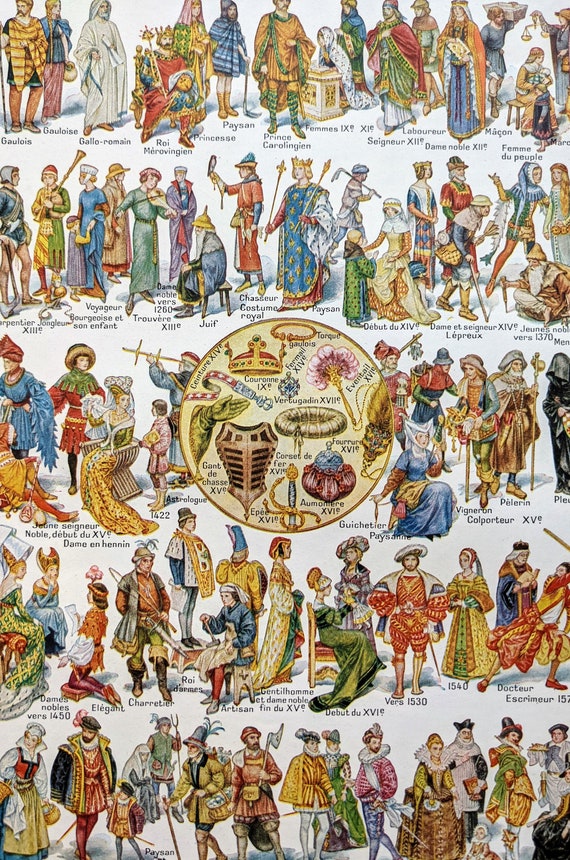This detailed illustration presents a bustling tableau of approximately 50 historical figures in diverse medieval and French-inspired attire. The image features five rows of characters, each clad in richly colorful garments ranging from royal gowns to armor, in hues of blue, red, orange, and yellow. Many figures possess accessories such as crowns, swords, axes, instruments, and canes, suggesting various roles from royalty to common folk, including kings, queens, jesters, and musketeers. The center of the piece is dominated by a yellow circle with a gold border containing detailed renderings of medieval accoutrements like a crown, armor, and the hilt of a sword. Each character is labeled with names in a non-English language using Arabic script, featuring titles such as 'artisan' and 'pelerin.' Despite the meticulous detail, some figures have disjointed features and proportion anomalies, hinting at possible AI generation. The overall composition resembles an intricate, educational art piece or poster designed to depict a vibrant historical panorama.